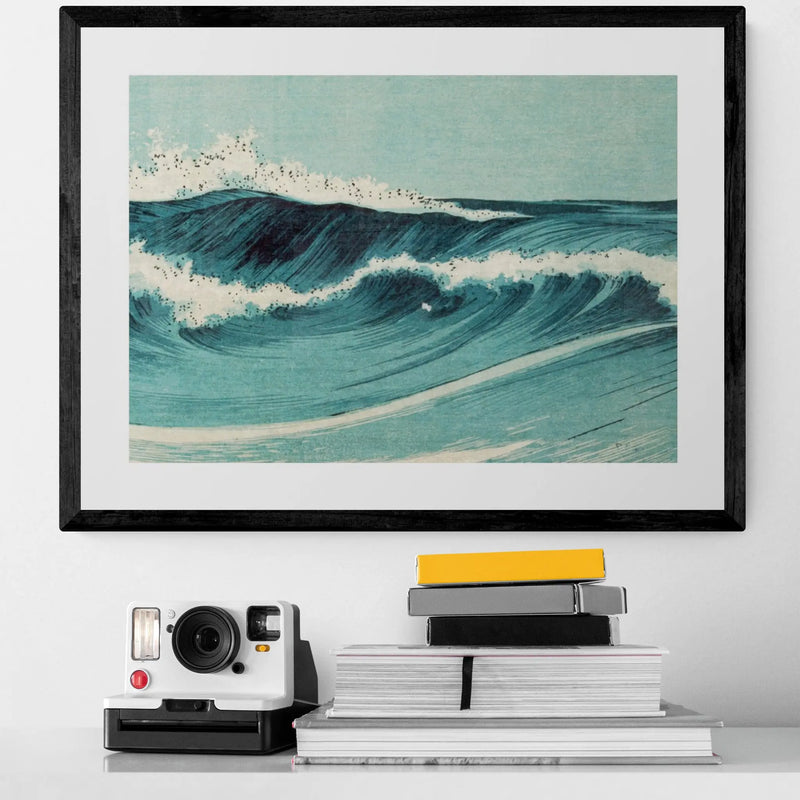This photograph captures a tastefully arranged desk against a white-painted wall, with a painting framed in black dominating the scene. The artwork depicts two large waves crashing downward, rendered in a light blue with darker blue streaks and white foamy crests speckled with black. The sky above these waves is a light blue with splotches of white, giving a serene yet dynamic feel. Below the painting sits a retro-style white Polaroid camera. The camera features a red flash button, a small square viewfinder to the right of the silver flash, an orange indicator light, and a cylindrical black lens. At the front, a black square slot marks where printed photos emerge. To the right of the camera lies a stack of books arranged by size, with the largest at the bottom and smaller ones on top. The books are in hues of gray, white, and possibly a mixture of other colors. At the very top of the stack rest three flat rectangular boxes, perhaps undeveloped Polaroid film, in black, gray, and Kodak yellow. The entire setup exudes a blend of modern decor mixed with nostalgic elements, creating a visually engaging and harmonious composition.